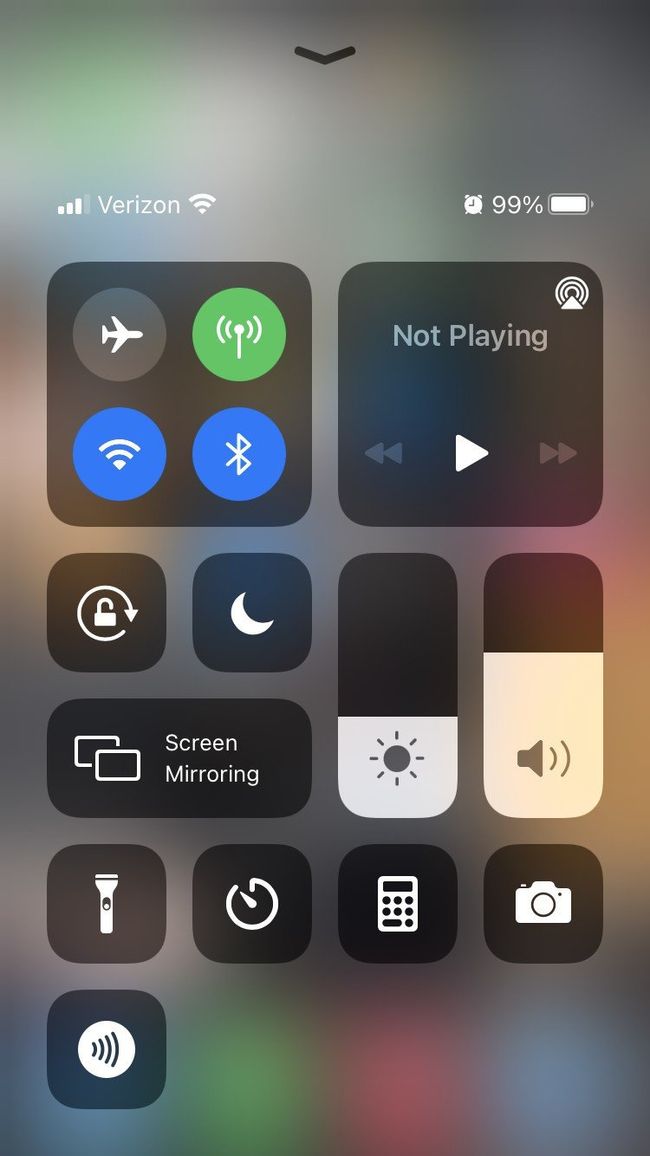This screenshot showcases the iPhone's Control Center, an essential utility menu overlay that appears over a blurred background of the main home screen. At the very top, a black arrow hints at the ability to swipe down to dismiss the menu. In this section, you'll see vital system information in white text: signal strength for the cellular network, the carrier name "Verizon," and Wi-Fi strength at maximum, symbolized by four bars forming a "V" shape. 

Adjacent on the right, an alarm clock icon is displayed, followed by a battery icon showing a 99% charge. 

The Control Center is segmented into 12 interactive icons. 

Top-left: The communication module includes toggles for Airplane Mode, Cellular Data, Wi-Fi, Bluetooth, and a signal indicator. 

Top-right: Here you'll find music playback controls and an AirDrop toggle. 

Middle-left: The screen orientation lock icon resides beneath the communication module, along with a crescent moon icon, likely indicating Do Not Disturb mode. 

Middle-right: Brightness and volume sliders allow for quick adjustments. 

Bottom-left: The Screen Mirroring icon facilitates projecting your screen to other devices.

Bottom row: Includes a flashlight, a timer, a calculator, and a camera icon, with an additional lone icon at the far right resembling a speaker, possibly indicating volume control or audio output options.

This extensive assortment of tools ensures swift access to essential iOS settings and functionalities.